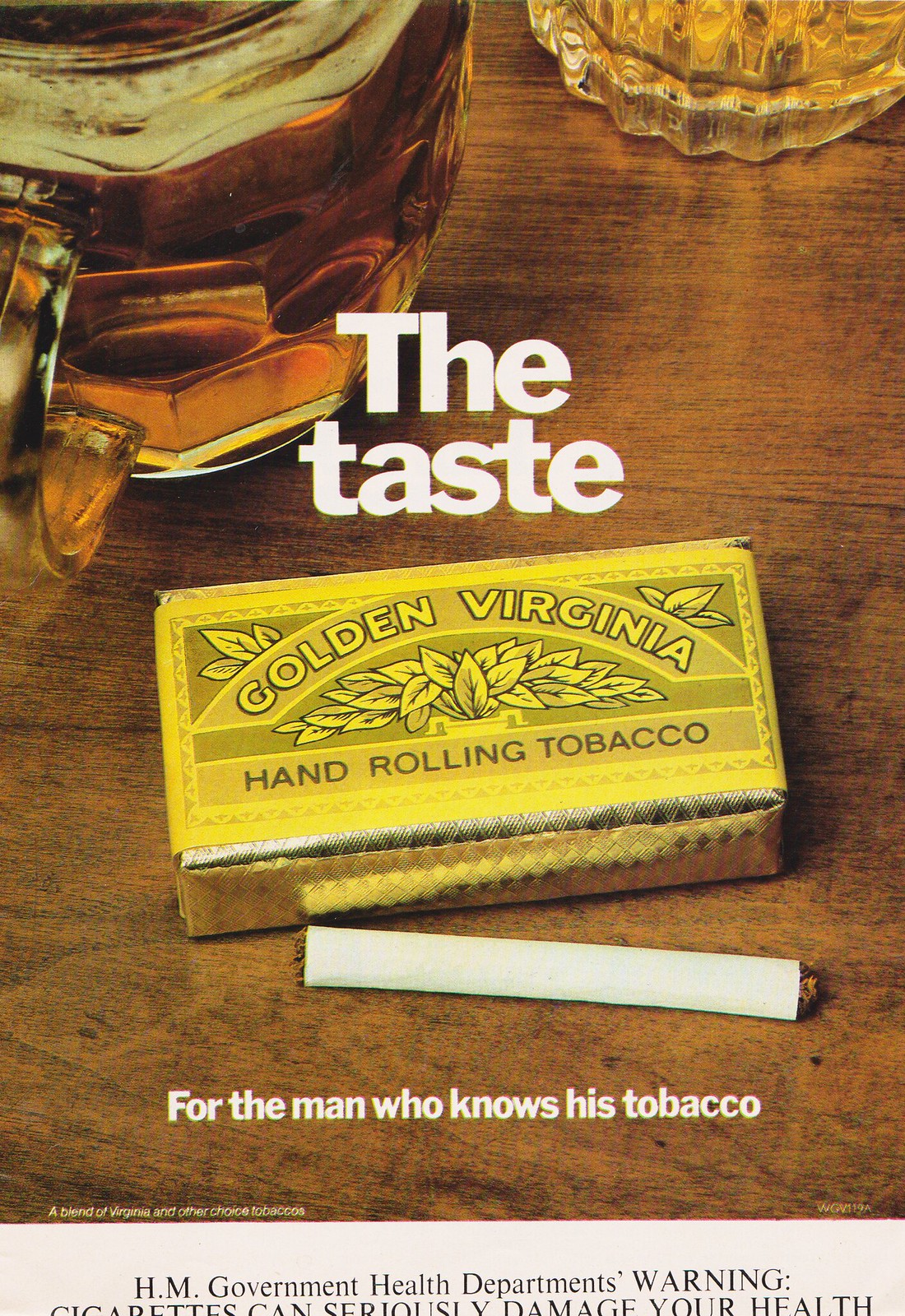The image is an advertisement for hand-rolling tobacco, prominently featuring a yellow box of Golden Virginia tobacco at its center. The box, adorned with an illustration of a tobacco plant, sits on a glossy brown wooden surface made up of horizontal boards. Above the box, large bold white letters declare "THE TASTE." Below the box, a rolled cigarette with visible brown tobacco peeking out is accompanied by the slogan "FOR THE MAN WHO KNOWS HIS TOBACCO." In the top left corner of the image, there is a clear glass cup filled with a brown liquid, possibly bourbon or beer, while the top right corner shows the lower part of another glass. The bottom part of the image transitions to a white background displaying a partially visible HM Government Health Department's warning, stating, "CIGARETTES CAN SERIOUSLY DAMAGE YOUR HEALTH."